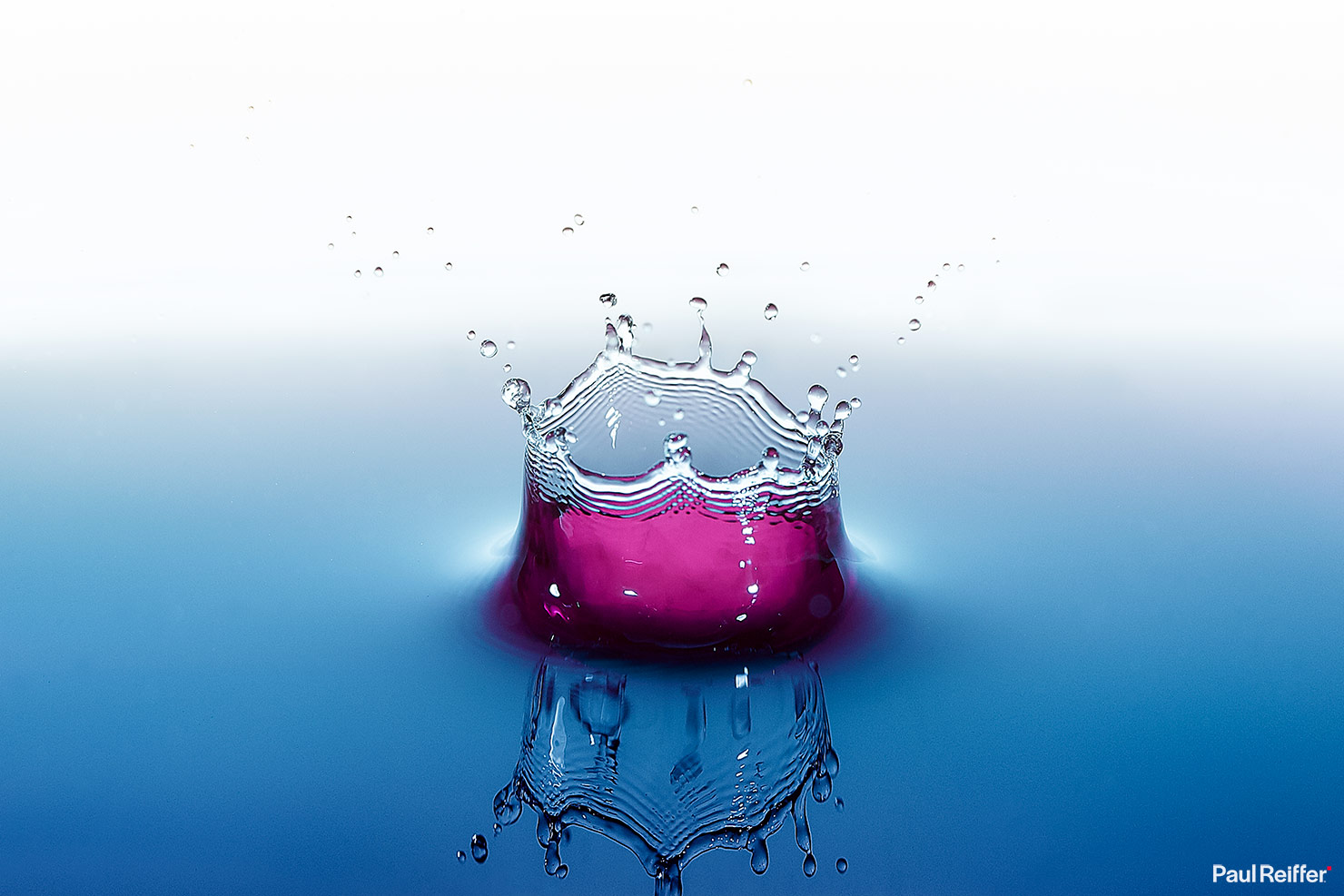A mesmerizing high-speed photograph captures the precise moment a droplet impacts the surface of the water, creating a stunning "crown" formation. The image features a gradient background, transitioning from pristine white at the top to a rich blue at the bottom, reminiscent of the meeting point between sky and ocean. The boundary between these colors is subtly blurred, enhancing the ethereal quality of the scene. In the lower right-hand corner, the signature "Paul Reiffer" marks the photographer's credit. The water droplet, rendered in a captivating pinkish-purple hue, rises majestically from the surface, its intricate crown-like shape mirrored perfectly below, adding a layer of depth and symmetry to the composition.